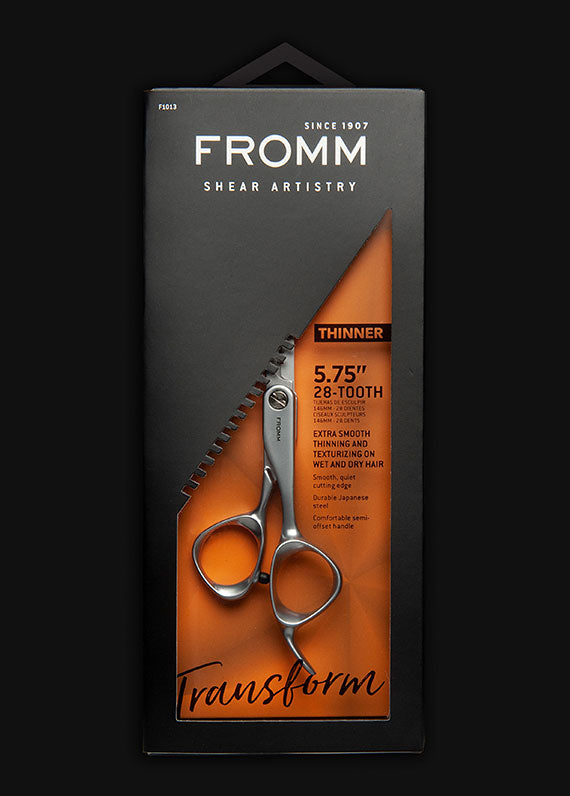The image features a meticulously crafted product shot against a solid black background, giving the product a floating effect. At the center is a black rectangular package showcasing a pair of high-quality hair thinning shears. The packaging, which measures around six inches tall and four inches wide, includes a hanger at the top for retail display, marked with the identifier "F1013." 

Prominent white text on the front reads, "Since 1907," followed by "Fromm Shear Artistry" in large capital letters, emphasizing the brand's long-standing expertise. Below the text, a razor-shaped cutout reveals an orange backdrop, providing a striking contrast against the silver shears inside. This cutout window, angled diagonally from left to right, features black text stating, "Thinner. 5.75 x 28 tooth," highlighting the specifications of the shears. Additional details indicate the shears' functionality: "Extra smooth thinning and texturizing on wet and dry hair," promising versatility and precision, while "Smooth, quiet cutting edge," and "Durable Japanese steel" emphasize quality and performance. At the bottom, the word "Transform" in script adds a final touch, suggesting the transformative capabilities of these premium shears.